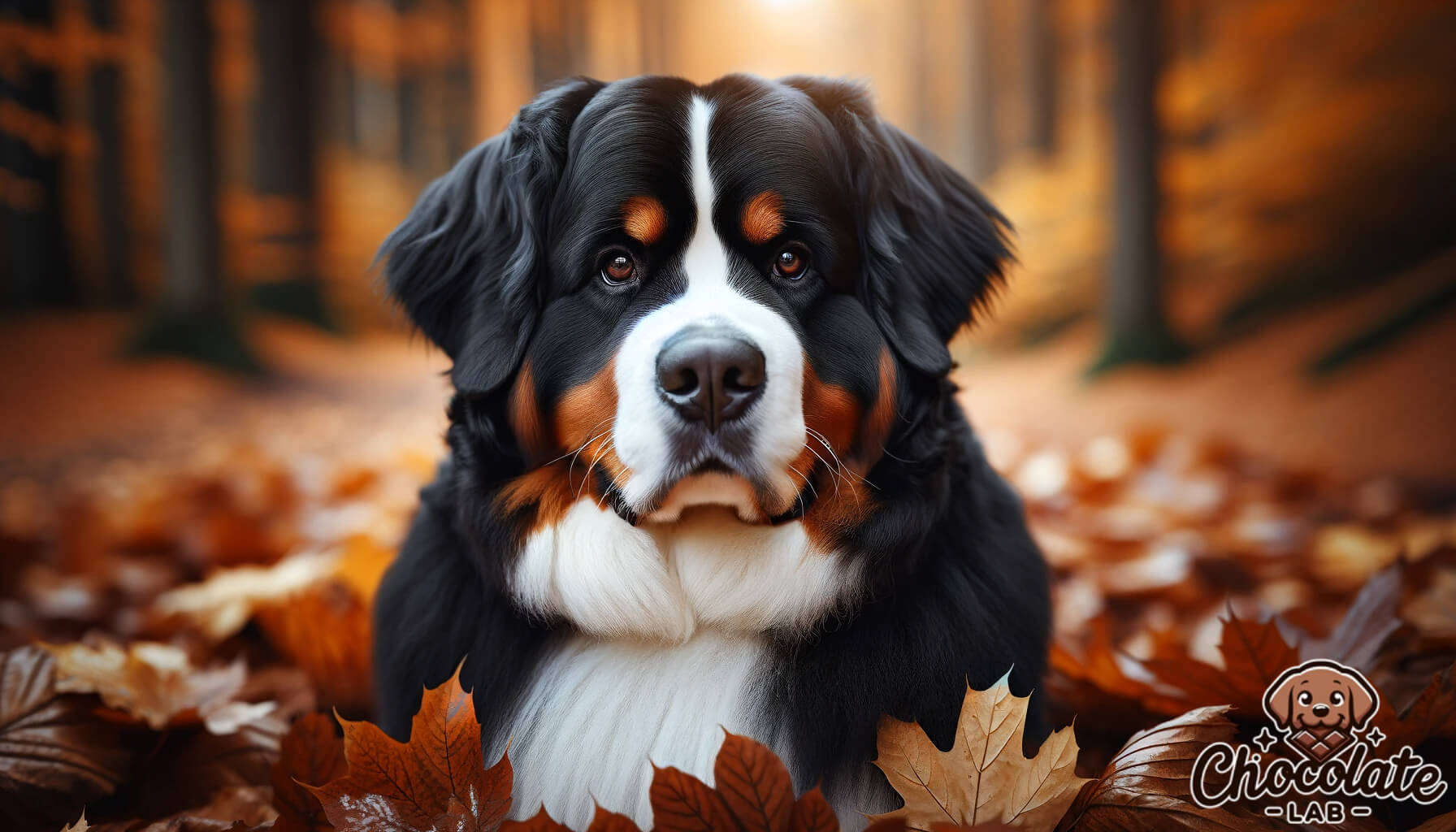In this detailed and visually stunning illustration, a majestic Bernese Mountain Dog sits prominently in the center of an autumn forest. The background is a blend of blurred oak and maple trees with a warm palette of oranges, browns, and blacks, resembling a beautiful painting. The forest floor is covered in detailed, crunchy fall leaves, adding texture and depth to the scene. The dog, with its striking black, brown, and white fur, has a wide head with big square ears, brown eyes, a white blaze down its front, brown cheeks, and a white chest. Despite its serious expression, the dog radiates a warm and inviting presence. In the bottom right corner, a charming cartoon logo features a little brown puppy with a piece of chocolate in its mouth and the text "Chocolate Lab," hinting humorously at either the breed or a fun play on words about a chocolate-making laboratory. This captivating image blends the beauty of nature with artistic creativity, making it a perfect piece of art worthy of admiration and display.